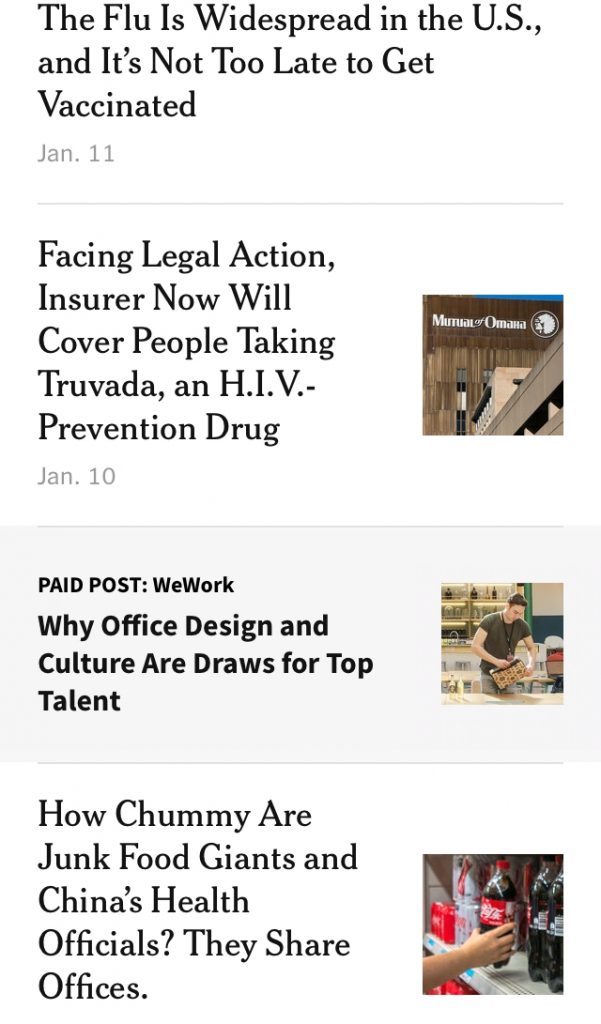This image captures a screenshot of a news website displaying four articles with the following headlines:

1. "The Flu is Widespread in the U.S. and It's Not Too Late to Get Vaccinated" dated January 11th. This article likely discusses the current flu season, emphasizing the importance of vaccination even if the flu is already widespread.

2. "Facing Legal Action, Insurer Now Will Cover People Taking Truvada, an HIV Prevention Drug." This piece covers a development where an insurance company, under legal pressure, has decided to offer coverage for the HIV prevention medication, Truvada.

3. "Paid Posts: WeWork. Why Office Design and Culture Are Draws for Top Talent." This sponsored article promotes WeWork, highlighting how their office design and company culture attract top-tier employees.

4. "How Chummy Are Junk Food Giants and China's Health Officials? They Share Offices." This investigative report delves into the close relationships between major junk food companies and health officials in China, pointing out that they even share office spaces. 

The image provides a snapshot of diverse topics ranging from public health issues and legal actions to corporate strategies and potential conflicts of interest in health regulation.